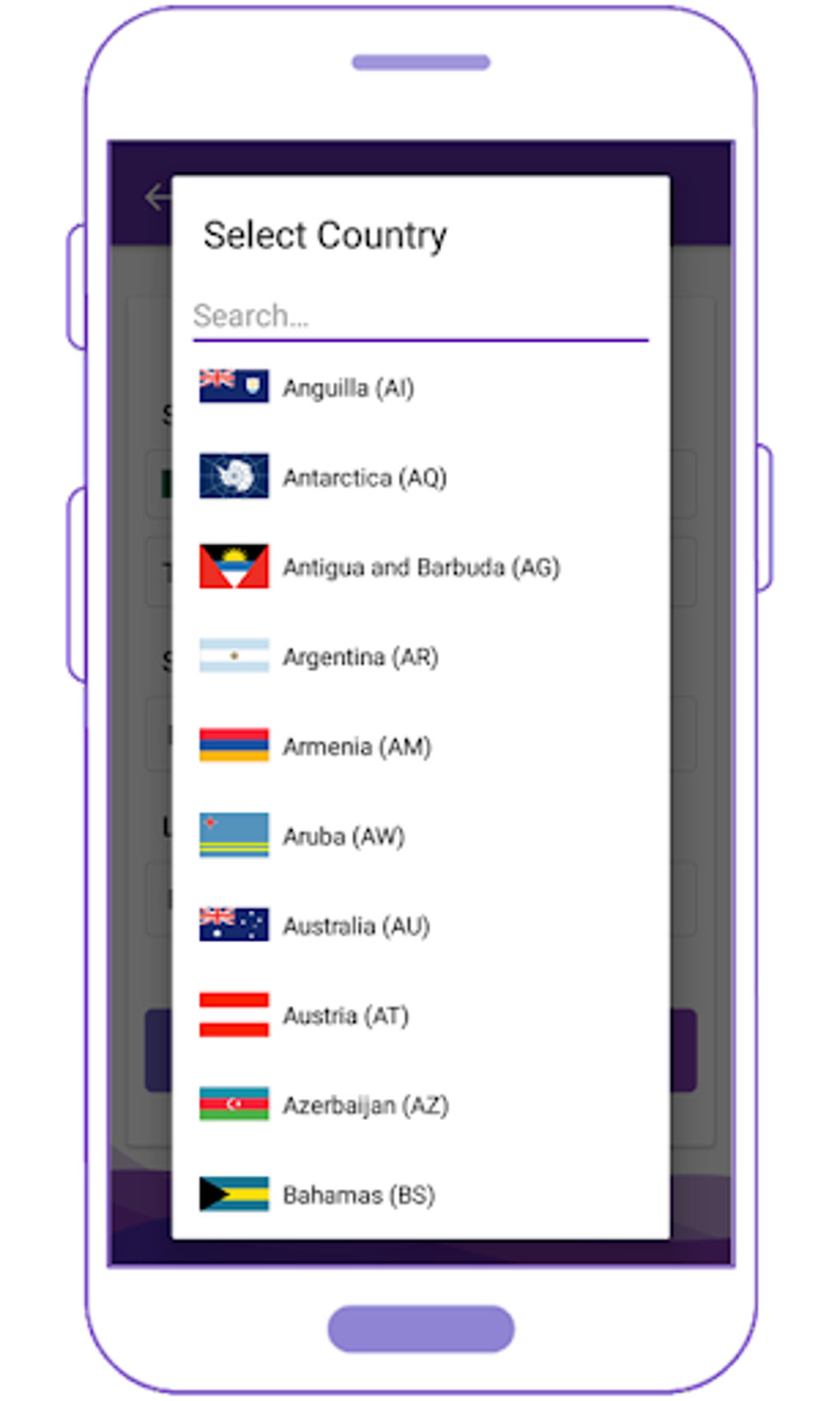A white Apple iPhone is prominently featured in the image, showing a screen with country search results. Among the listed countries are Texas, Anguilla, Antarctica, Antigua and Barbuda, Argentina (AR), and Armenia (AM). The screen also displays Nuba (IW), Australia, Austria (featuring red-white-red flag colors), Azerbaijan, and the Bahamas. The back of the smartphone is visible, with a blurred background creating an out-of-focus effect that enhances the subject. The edges of the phone have a purple hue, forming a slightly purple oval shape. The sides of the iPhone include gray buttons on both the left and right edges. This high-resolution image captures the elegance of the smartphone while highlighting the variety of flags associated with different countries.